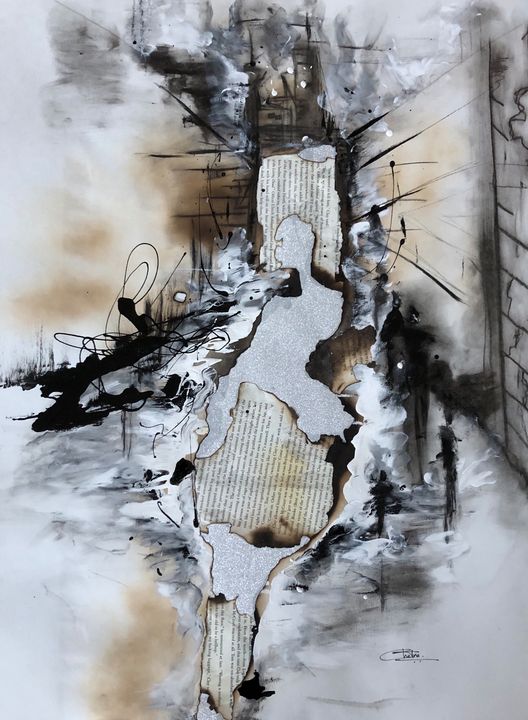This intriguing and modern artwork features a highly abstract and intense composition that primarily involves burnt pieces of paper. These fragments appear to be torn from a book or newspaper, exhibiting irregular, charred edges with some legible text showing vertically, though the words remain indecipherable. The burnt paper is centrally positioned and is surrounded by chaotic, expressive black, white, and gray designs that resemble clouds, smoke, ink, and ash, creating an explosive and dynamic visual effect. The background includes lighter hues such as silver and hints of dark brown, contributing to the burnt, smoky atmosphere. This multimedia piece, signed in dark ink in the lower right corner, incorporates intricate textures and layers, exemplifying an abstract and intense artistic expression.